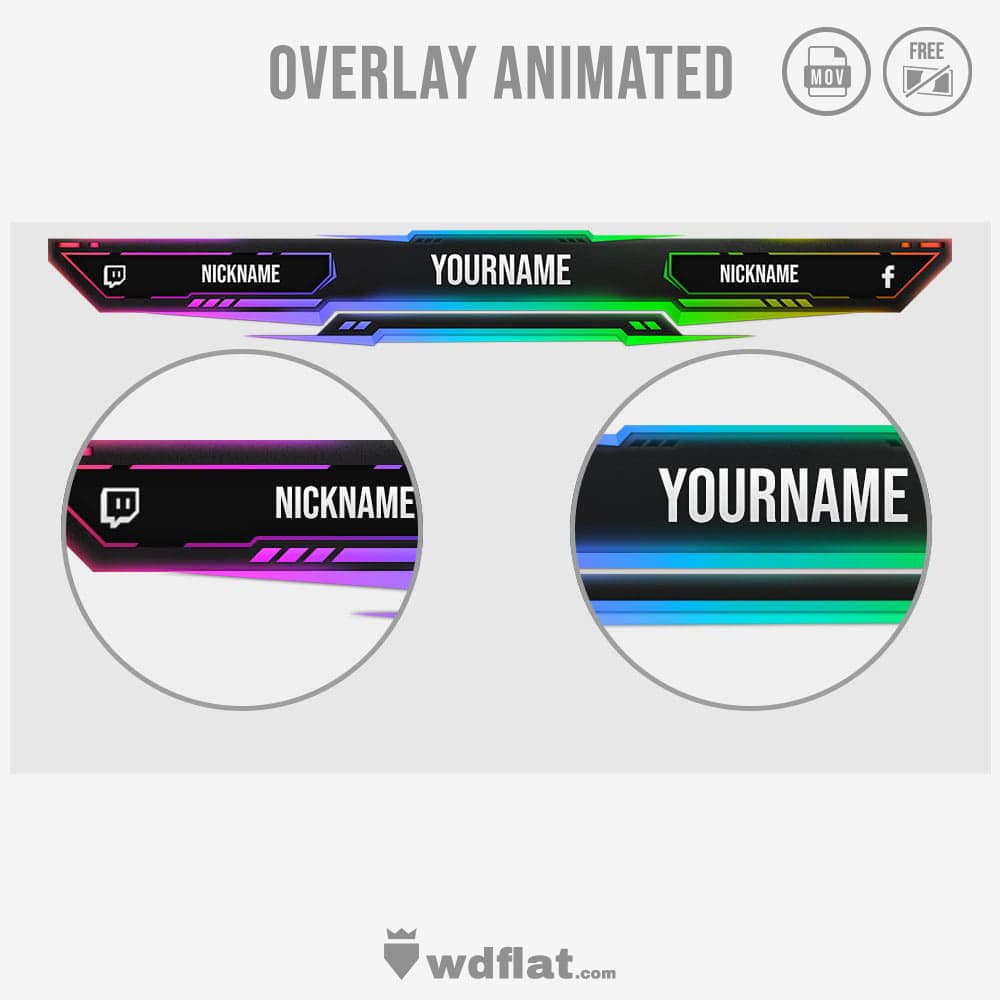This collar advertisement is set against a white background and prominently features the text "overlay animated" at the top. The design includes two circles near the top: the left circle resembles a notebook piece of paper and is marked "M.O.B.", while the right circle, labeled "free," has a computer screen icon with a slash through it, indicating an excluded ingredient. The vibrant color scheme includes neon shades of blue, green, orange, purple, and pink, making the item stand out.

In the center of the advertisement, the words "your name" are displayed, flanked by "nickname" on both the left and right sides. Additionally, a Facebook symbol is positioned on the far right. Below this central text, there are two magnified, blown-up views of the "nickname" text on each side.

At the bottom of the poster, there's an emblem featuring a crown within an upside-down triangle along with the website "WDflat.com." The overall design is modern and eye-catching, utilizing bright neon colors to draw attention.